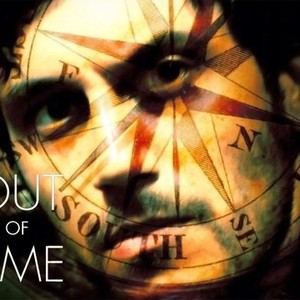This color photograph captures a close-up of a man’s face overlaid with the imagery of a red and black sundial-compass hybrid. The man's dark hair, which frames his face at about mid-length, blends into the black background. His left eye forms the center of the sundial, which fans out with star-like points indicating various directions such as North, South, and Southeast. The sundial’s intricate design adds layers of meaning to his stern and concerned expression. He is slightly unshaven, with a prominent afternoon shadow that enhances his rugged appearance. A partially cut-off white text appears in the lower left corner, with only the letter "M" visible, suggesting it might be the word "time." The man’s head is slightly tilted to the left, and he sports a mustache and sideburns, further contributing to his intense, contemplative visage.